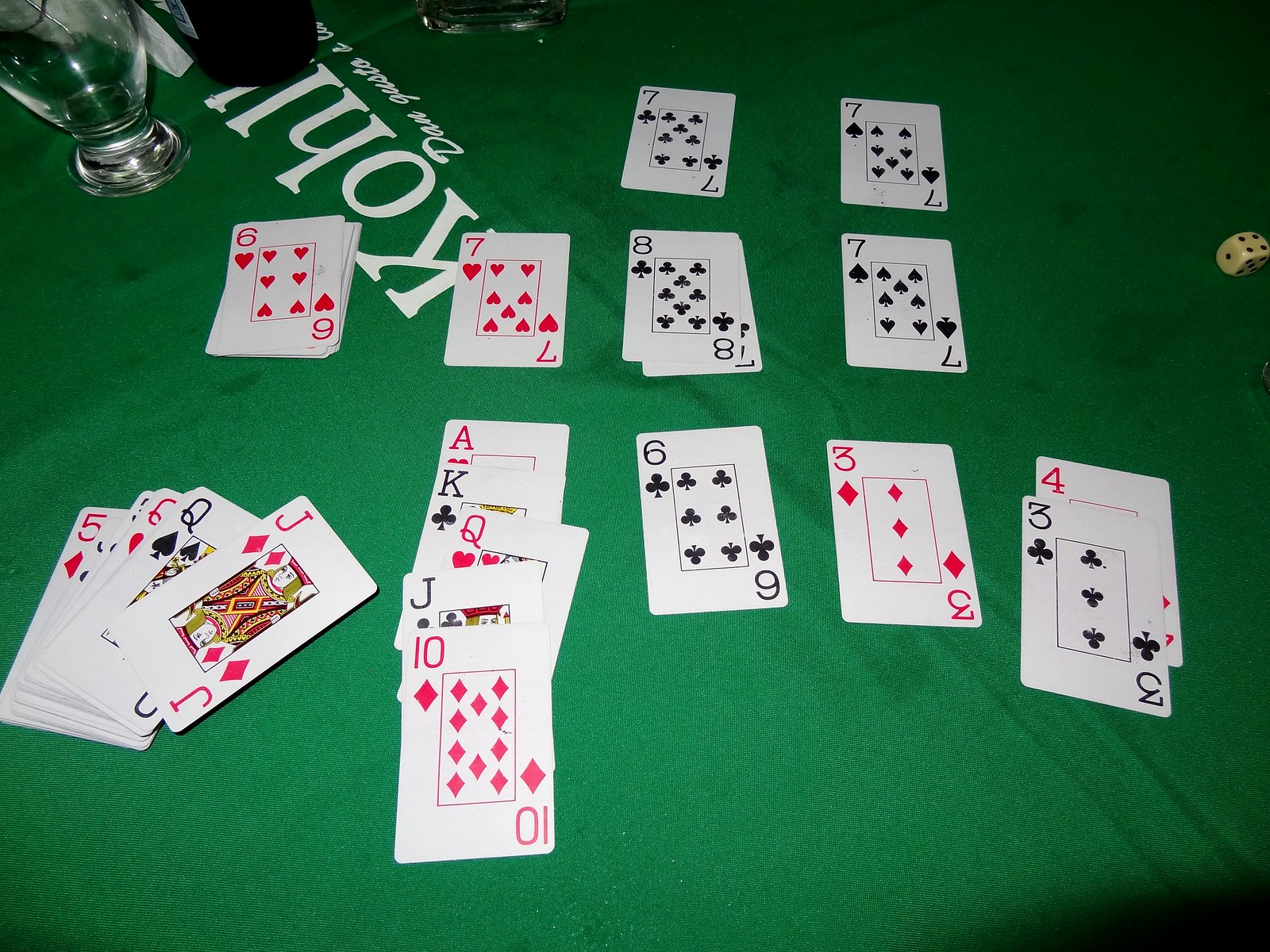The image showcases a detailed layout on a green card table. Various playing cards are meticulously arranged:

- In the top right corner, there's a seven of spades.
- To the left of the seven of spades is a seven of clubs.
- Underneath the seven of clubs lies an eight of clubs.
- To the immediate right of the eight of clubs is a seven of spades again.
- Below this seven of spades is a three of diamonds.
- To the right of the three of diamonds is a three of clubs.
- Next to the three of clubs is a four of diamonds.
- To the left of the three of diamonds is a six of clubs.
- Directly above the six of clubs is another eight of clubs.
- Further left of the eight of clubs is a seven of hearts.
- Two cards to the left of the seven of hearts is a six of hearts.
- Below the seven of hearts is an ace of hearts.
- To the right of the ace of hearts is a king of clubs.
- Following the king of clubs to the right is a queen of hearts.
- Next to the queen of hearts is a jack of clubs and then a ten of diamonds.
- To the left of the ten of diamonds is a jack of hearts.
- More cards appear to be stacked and hard to read in the lower sections of the table.
- On the far left side of the layout is a five of diamonds.

Additionally, on the far right side of the table, a die shows the number four. A drinking cup is positioned at the top left of the table. The entire setup hints at a game in progress or ready to begin on a vibrant green gambling table.